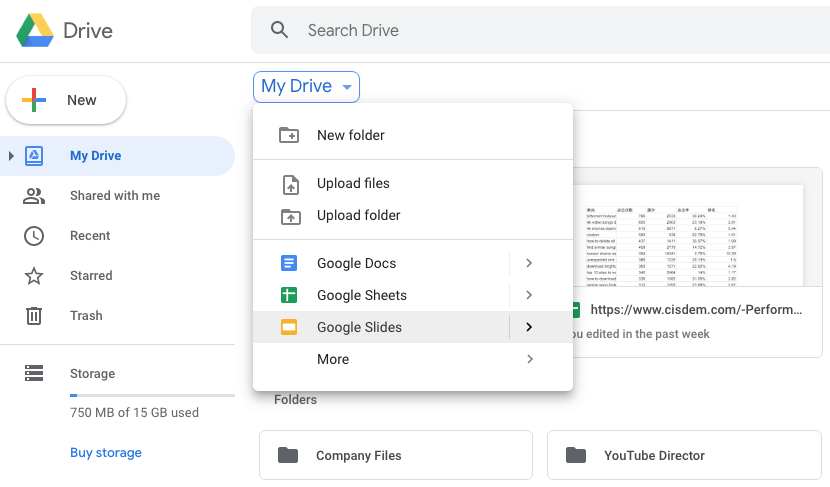This screenshot is a cropped view of the Google Drive interface. It prominently displays the Google Drive icon at the top left corner, adjacent to a search box labeled "Search Drive." On the left side, a vertical panel contains various options capped by a circular "New" button with a plus icon. Below this button, the options listed are My Drive, Shared with Me, Recent, Starred, Trash, and Storage, with "My Drive" highlighted in blue, indicating its selection.

A pop-up menu is visible toward the right side of the panel, presenting file management actions such as "New Folder," "Upload Files," "Upload Folder," "Google Docs," "Google Sheets," and "Google Slides," with "Google Slides" currently selected. 

In the central part of the screenshot, partially obscured by the pop-up menu, there is a document that has been recently edited. The bottom right corner displays large boxes titled "Company Files" and "YouTube Director." At the bottom left, small blue letters read "Buy Storage." The overall background of the interface is white.